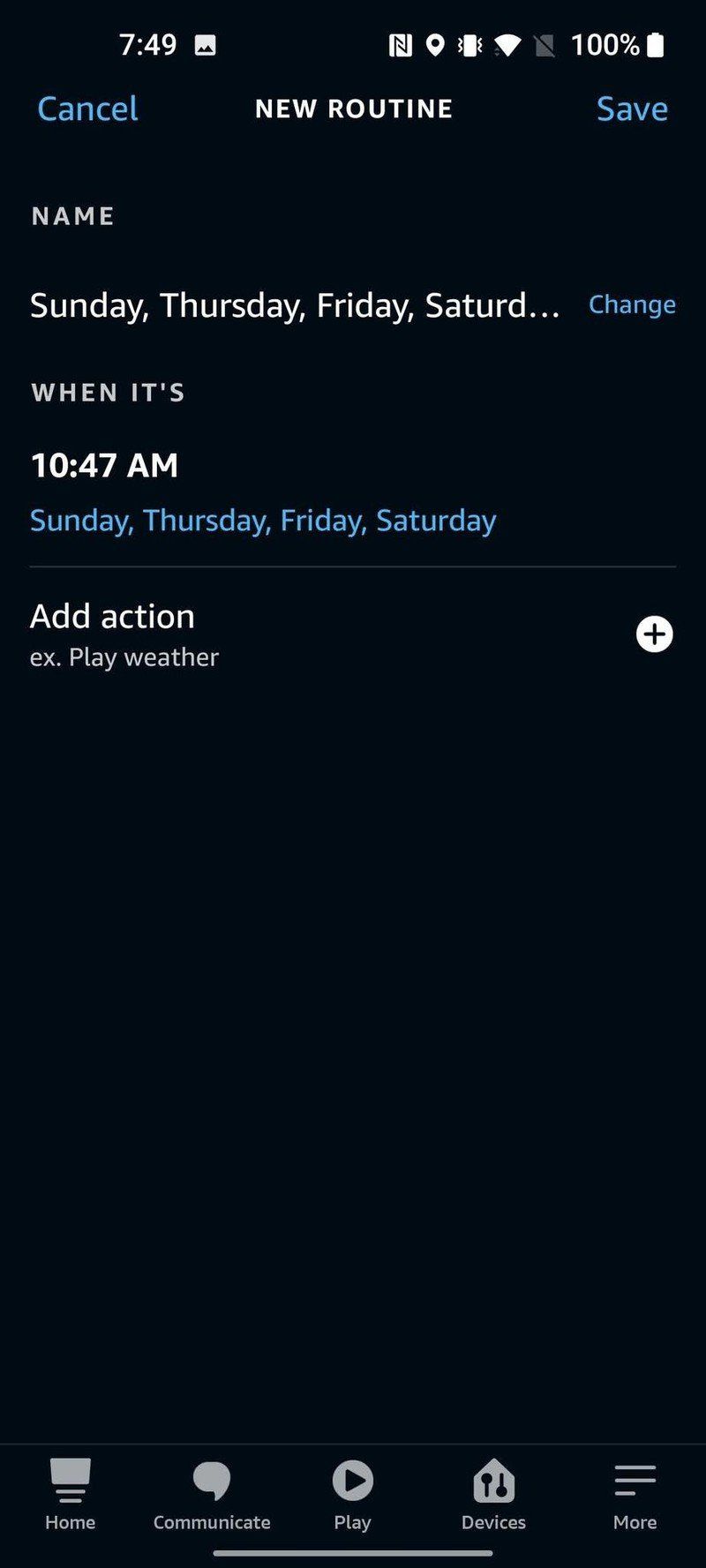Detailed Caption: 

The image showcases a smartphone screen displaying an app interface against a navy blue background. At the bottom of the screen, there are five semi-white, somewhat gray icons representing different functionalities. Starting from the left, the icons include: a 'Home' icon, a 'Communicate' icon depicted as a thought bubble, a 'Play' icon resembling a video play button, a 'Devices' icon illustrated as a house with an up and down switch, and a 'More' icon shown as three horizontal lines.

At the top of the screen, the time is displayed as '7:49' in white text, alongside an images icon. In the upper right corner, several status indicators are visible: an 'N' inside a white box, a GPS pinpoint icon, a vibration icon, and indicators for data/Wi-Fi, a crossed-out SIM card, a battery at 100% charge, and a fully charged battery icon.

Below this, the screen displays options to 'Cancel' (on the left) and 'Save' (on the right, highlighted in blue) with 'New Routine' in white text centered between them. The routine seems to be labelled 'Name' with days of the week listed as 'Sunday, Thursday, Friday, Saturday.' There’s also an option marked 'Change When It's' with a specified time of '10:47 AM' for 'Sunday, Thursday, Friday, Saturday.' Additionally, there's an 'Add Action' section featuring an example prompt to 'play weather,' accompanied by a plus icon for adding actions.